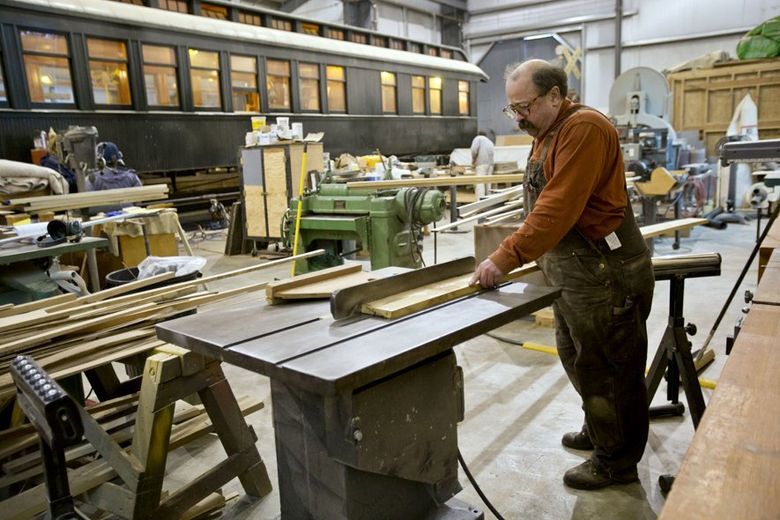This is a color photograph of a balding, heavyset man with brown hair, glasses, and a thick mustache, working in an industrial woodworking shop with gray and white walls, illuminated by fluorescent lighting. He is wearing a long-sleeved brown shirt, dark dusty overalls, and black work boots. The man stands on a concrete floor at a workbench, pushing a piece of wood through a metal-colored saw. The workshop is filled with various woodworking tools, machinery, and numerous piles of wood, including a green machine in the middle of the floor. Along the right side of the image, there are brown desks and workbenches. In the background, to the left, there is a large dark brown or black bus or train car with lights on inside and several windows, adding to the cluttered, industrious atmosphere of the scene.